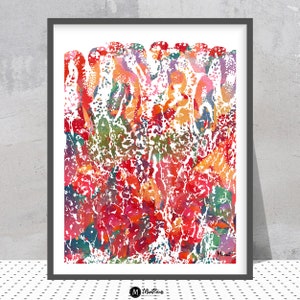The image features an abstract painting framed in a sleek black frame with a white border and is leaning against a gray wall. The painting itself is a vivid array of colors including shades of red, orange, pink, purple, green, and blue, displayed in a modern, non-representational style. While the depiction within the frame is open to interpretation with circular and oblong shapes, some viewers see potential figures, perhaps abstract forms of penguins or other entities. The frame's shadow is cast to the bottom right, adding depth to the composition. The frame rests upon a white surface adorned with black polka dots, grounding the scene. A difficult-to-read watermark is located at the bottom center of the image, hinting at the print's possibly commercial nature.